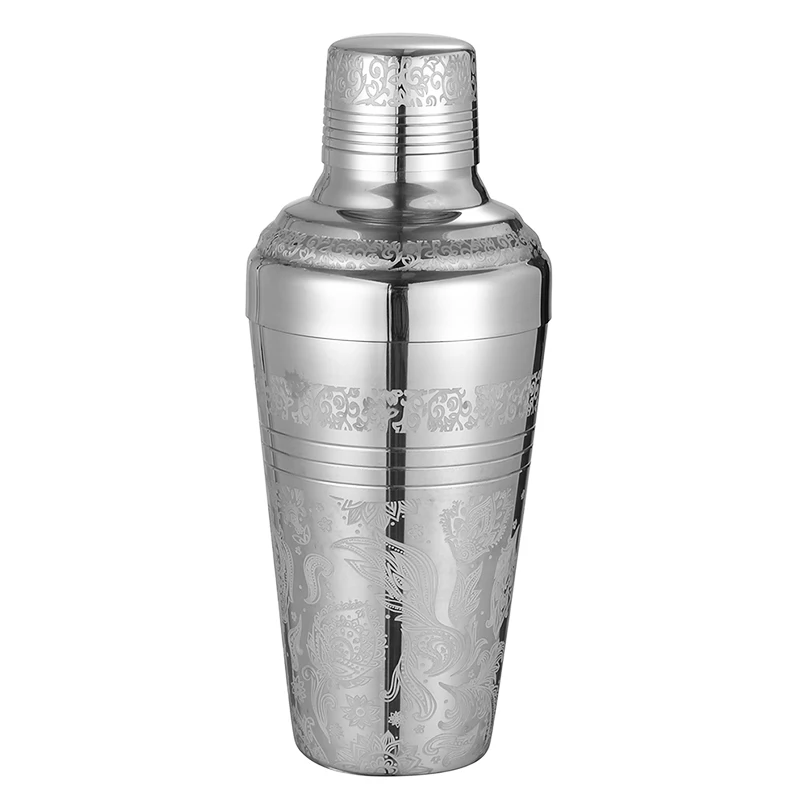This photograph captures a tall, shiny silver container placed against a pure white background. Shaped similarly to both a decorative urn and a cocktail shaker, the container narrows at the base, widens gradually towards the shoulders, and then tapers again towards the cap. The cap itself features horizontal striping, consistent with the rest of the item's metal construction and possibly indicating a screw mechanism.

Intricate etchings adorn the container, including three parallel horizontal bands of floral spiral designs around the middle to the upper portion. The lower part of the container is embellished with swooping abstract patterns reminiscent of flowing fish fins, while the floral motifs include curvy designs with flower bulbs and many intricate leaves. The filigree work is very detailed and reflective, showcasing the metallic finish.

Light reflects off the object's surface, enhancing its shiny appearance, and a vertical black stripe can be seen running down the middle from the cap to the base. The image, likely intended for product showcasing, emphasizes the container's elaborate detailing and polished silver finish.